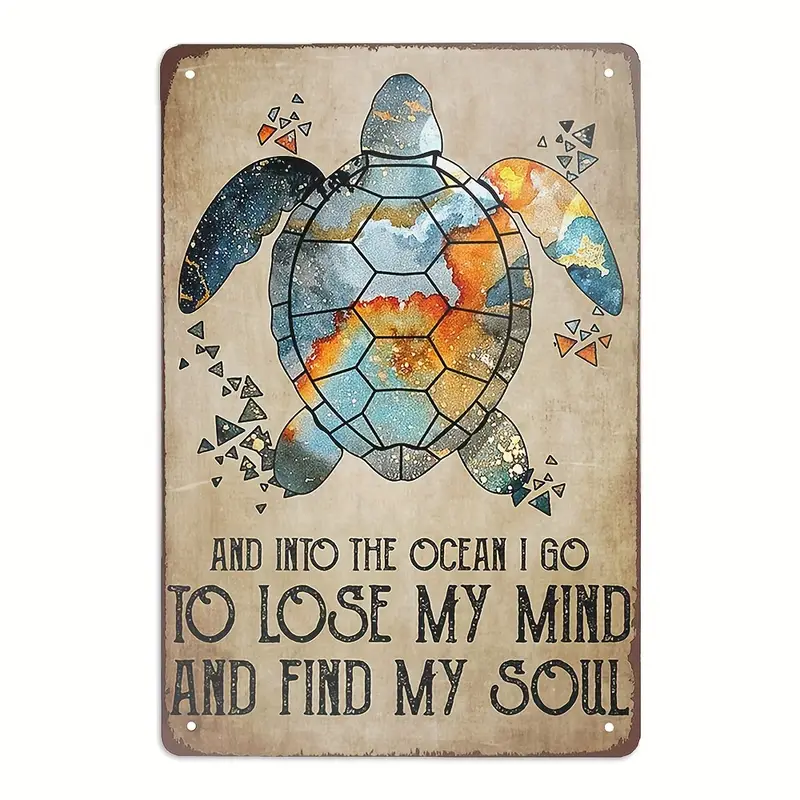The image depicts a worn, vintage sign with small holes in each corner, indicating that it was likely hung up at some point. The sign's background is a weathered tannish gray color. The central feature of the image is a large sea turtle, which is multicolored, displaying hues of green, orange, yellow, red, blue, and gray. The turtle appears to be lying on its stomach with its four legs spread out, and its paint is slightly faded and chipped, suggesting it has been exposed to the elements. Surrounding the turtle are additional triangular-shaped objects in various colors. Below the image of the turtle, there is a motivational quote in black text that reads: "And into the ocean I go to lose my mind and find my soul." The overall style of the piece is that of a motivational poster or plaque, designed to inspire and resonate with its viewers.